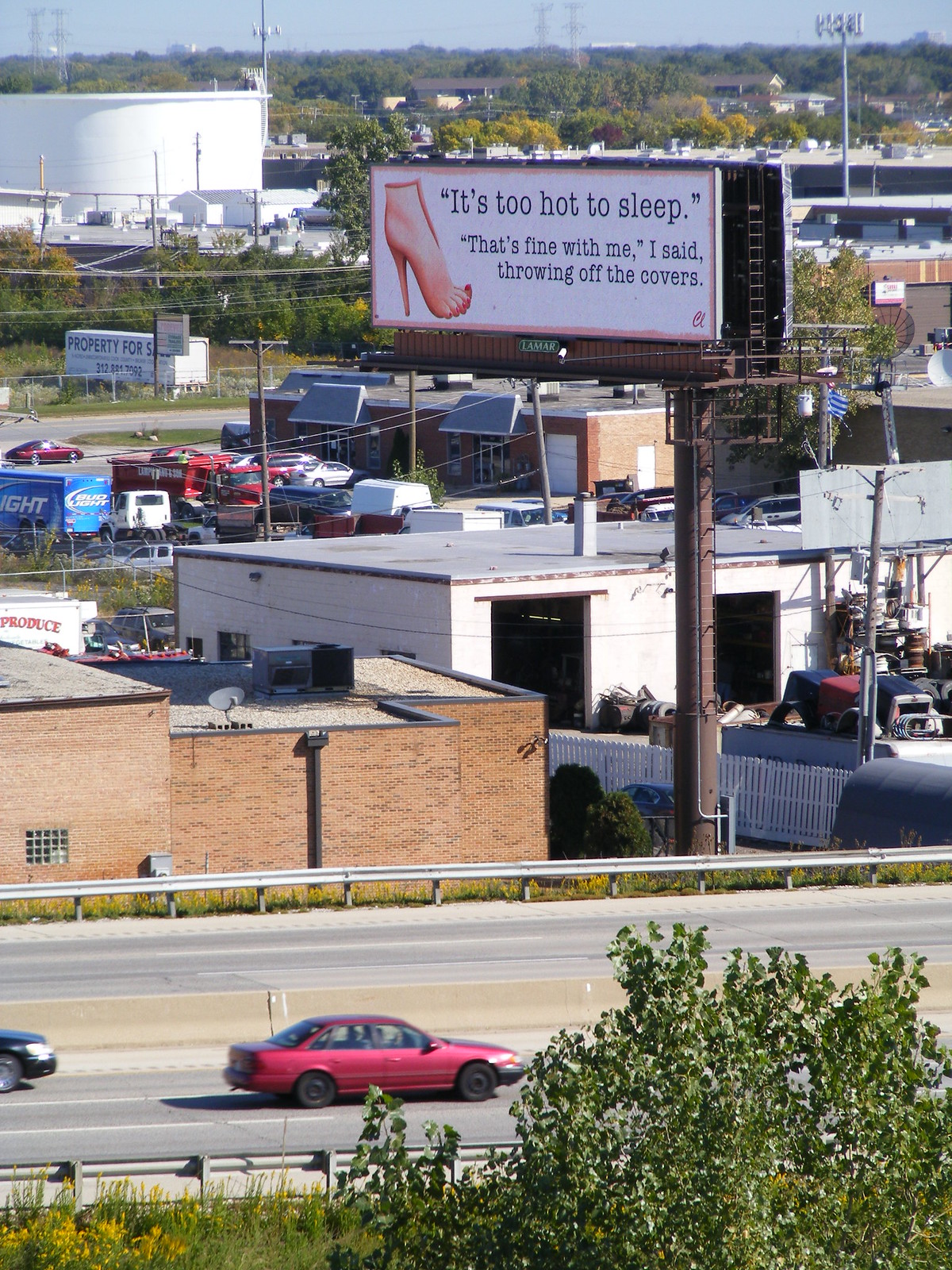The photograph captures a vibrant, industrial downtown area viewed from an elevated vantage point on a bright, sunny afternoon. In the foreground, a busy three-lane highway features a red sedan in motion, with a black car following closely behind, partially cut off by the edge of the image. A concrete divider separates the traffic lanes. Off to the left, we catch a glimpse of a dark blue or possibly black vehicle. 

Dominating the center of the image is a large white billboard, mounted on a rust-colored steel pole. The billboard features a detailed illustration of a woman's bare foot with elegantly curled toes painted red, adorned with a very thin red ankle strap and a delicate strap between the big toe and the others. A flesh-colored, pointed heel extends from the foot, creating a striking visual. The billboard's text in black reads, "It's too hot to sleep." Following this are the words, "That's fine with me, I said, throwing off the covers."

In the background, a series of industrial buildings can be seen, including a brown brick structure and a white building with two large garage bays and a grey roof, surrounded by old parts. Semi-trailers, including a blue Bud Light truck, are parked in various spots. Surrounding the area are multiple brown buildings and an expanse of trees under a clear blue sky. Power lines traverse the scene, adding to the industrial ambiance.